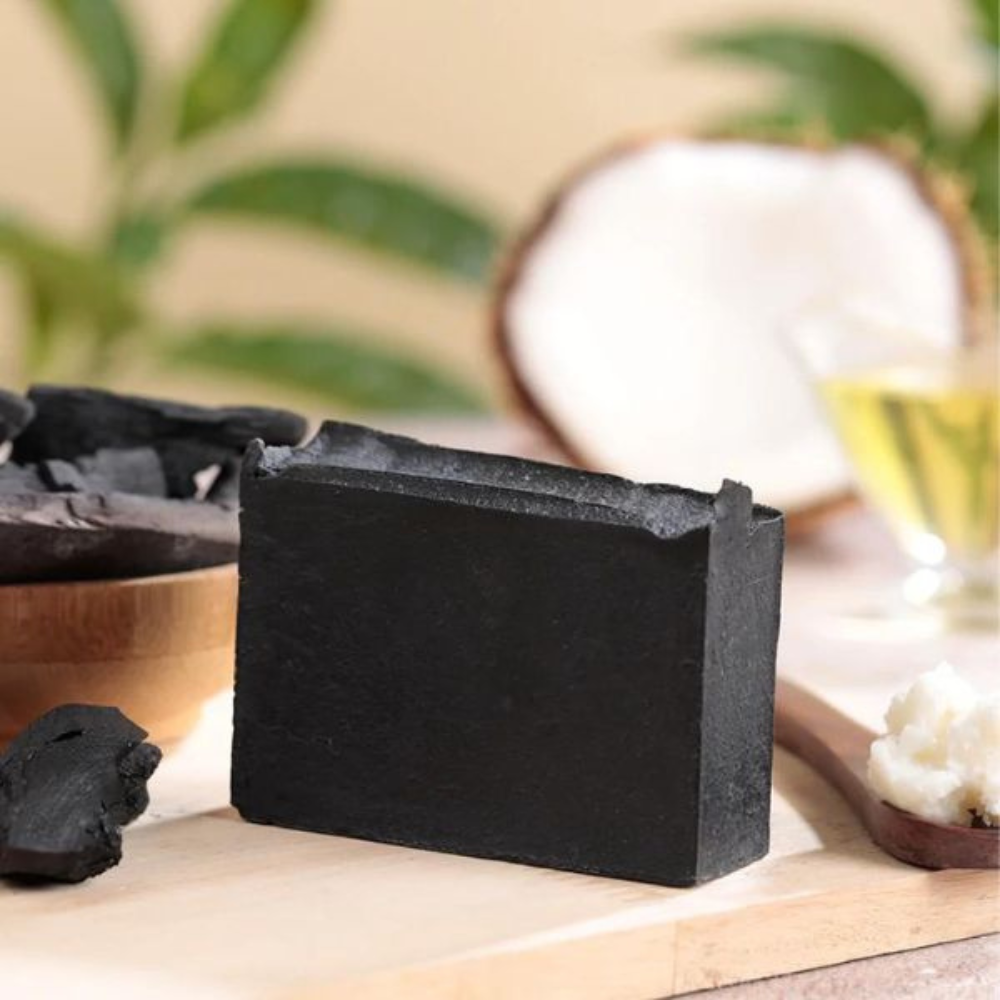The image vividly captures a rustic scene centered around a rough-looking tabletop. Positioned diagonally across the table is a 2x4 plank, which serves as a base for various objects. The most prominent is a black square object resembling a charcoal block, positioned near the center of the image. To its left, there's a smaller piece of charcoal, and to its right, rests a wooden spoon containing a white substance.

In the background, the details are noticeably blurred but reveal the hints of green foliage and a wall. Additional items in the scene include a cup with a golden liquid on the right, possibly wine or champagne, and a partially visible coconut shell. On the left, there is a brown bowl containing more pieces of charcoal. The image is devoid of text and showcases a warm color palette featuring tan, green, brown, white, yellow, off-white, light brown, black, and beige. Despite the blurred background, the intricate foreground details stand out, making it unclear whether the photo was taken indoors or outdoors, though it suggests a daytime setting. The photograph is taken at eye level, focusing on the central charcoal block and the surrounding rustic elements.